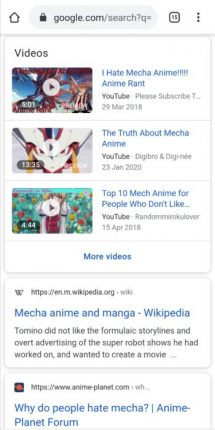This image, taken from a Google search results page, showcases previews for three videos related to the topic of MECHA anime. 

The first video is titled "I HATE M-E-C-H-A-N-I-M-E!!!" and comes with a caption urging viewers to subscribe to the YouTube channel. It was uploaded on March 29, 2018, and has a runtime of 5 minutes and 1 second. The preview image features a play button centered over a visually striking background of red, blue, and white graphics.

The second video, titled "The Truth About M-E-C-H-A-N-I-M-E," is presented by Digibro and Digi-Knee. Uploaded on January 23, 2020, this video lasts for 13 minutes and 35 seconds. The thumbnail features an anime graphic with prominent white, red, and yellow colors.

The third video, "Top 10 M-E-C-H-A-N-I-M-E for People Who Don't Like YouTube," is uploaded by Random Roku Lover and dated April 15, 2018. It has a runtime of 4 minutes and 44 seconds. The preview image displays an anime lady set against a backdrop of green, red, and yellow floral graphics.

Below the video previews, there are options to view more videos and links to further resources. These include a link to a MECHA Anime and Manga Wikipedia page and another to a discussion titled "Why Do People Hate M-E-C-H-A?" on Anime-Planet forums, found at www.anime-planet.com.